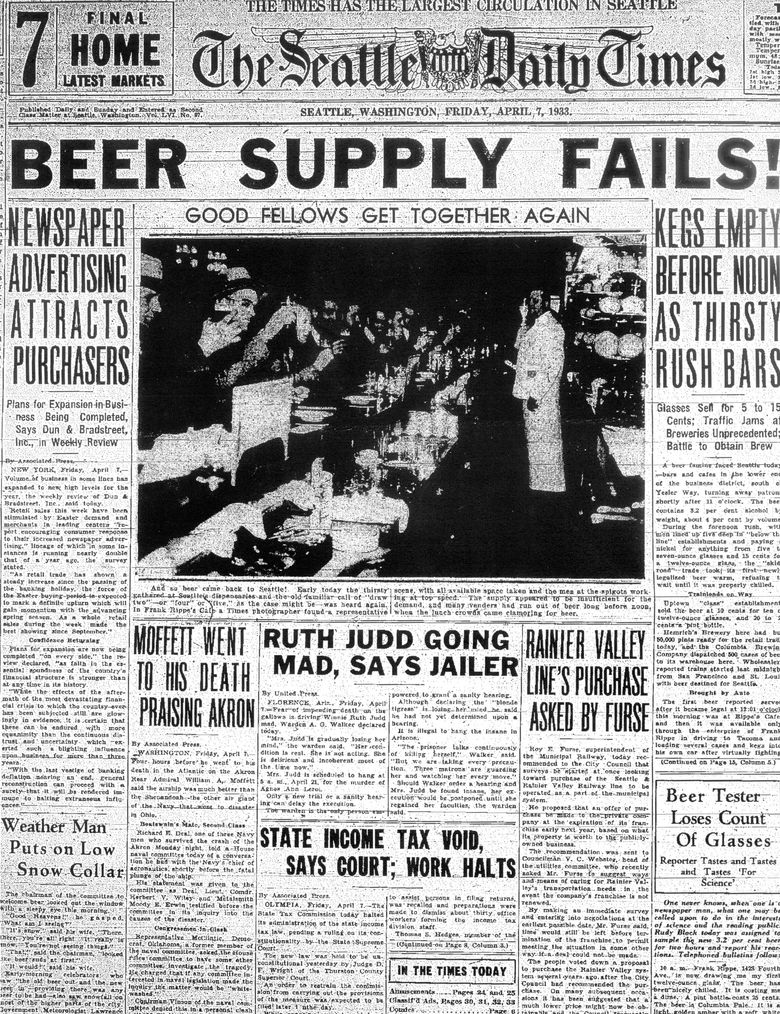The front page of the **Seattle Daily Times** dated **Friday, April 7th, 1933**, is presented in a **black and white photograph**. The dominant headline reads in bold, capital letters, "BEER SUPPLY FAILS!" stretching the full width of the page. Just below this headline, there’s a subheader in all capital letters, "GOOD FELLOWS GET TOGETHER AGAIN," accompanied by a black and white photo of a group of men gathered at a bar. 

In the image, a man dressed in white, possibly a server or chef, stands behind a counter, attending to patrons who appear to be enjoying their drinks. Their attire suggests they are from an earlier era, potentially the 1930s, consistent with the date of the newspaper.

Surrounding the central image and headline are various smaller articles and captions such as "Newspaper Advertising Attracts Purchasers," "Kegs Empty Before Noon as Thirsty Rush Bars," and "Beer Tester Loses Count of Glasses." Other readable headlines include "Ruth Judd Going Mad Says Jailer," "Rainier Valley Lines Purchase Asked by P.U.D.," "State Income Tax Void Says Court Work Halts," and "Weatherman Puts on Low Snow Collar." 

The page is filled with dense text in smaller print, capturing the reader’s attention with its myriad of news stories and updates, all framed by the central, larger headline and accompanying photograph.